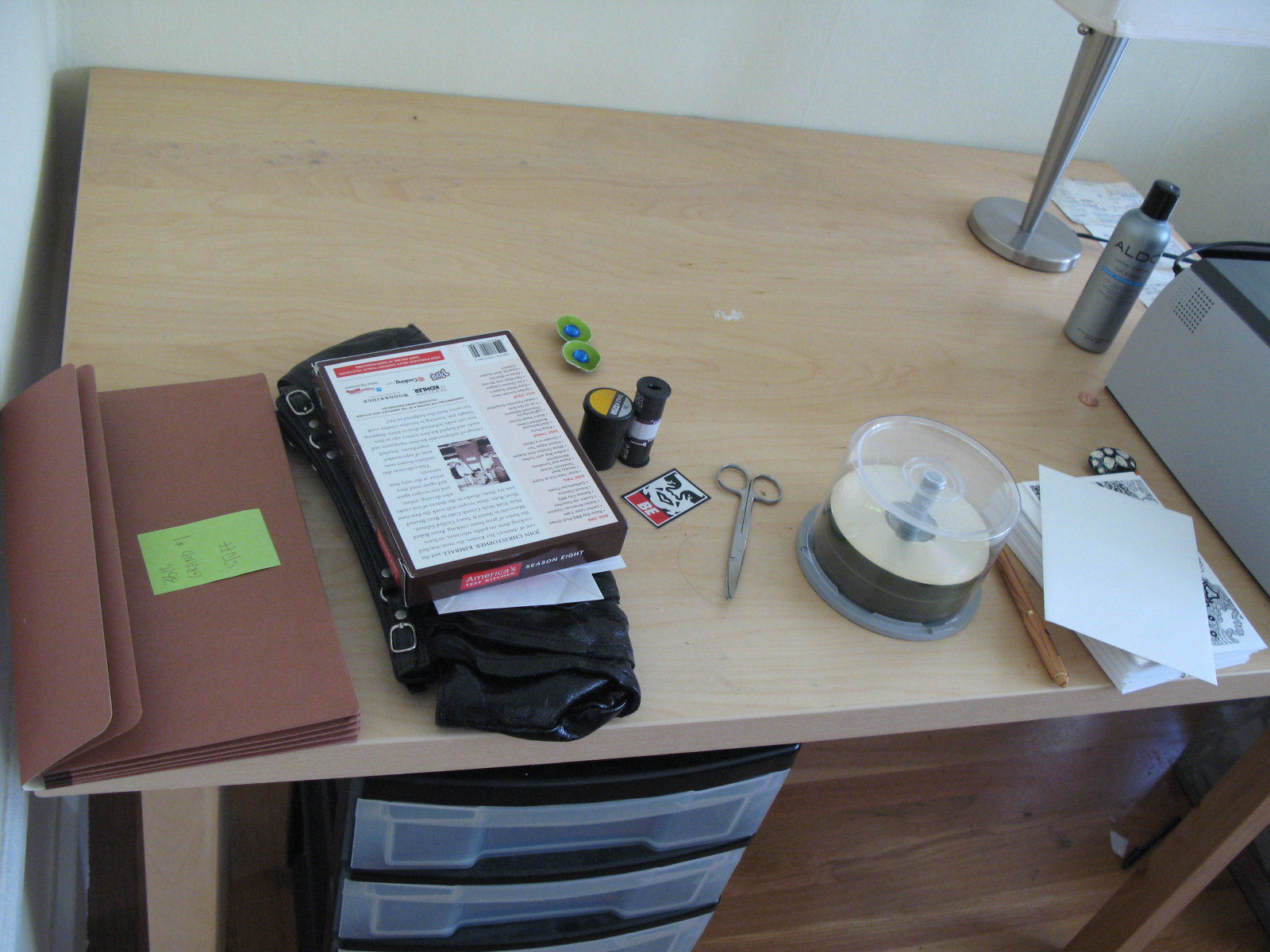A top-down view captures a wooden table positioned on a slightly darker hardwood floor. Underneath the table, there is a plastic storage container with white drawers, providing hidden storage. On the table's surface rests a black, folded woman's purse, which holds a DVD case atop it. Adjacent to the purse, a brown file holder lies flat. To the right of the purse, a pair of scissors is neatly placed alongside two spools of thread. Completing the assortment of items is a black, transparent glass case that houses several DVDs, contributing to the organized yet busy scene on the table.